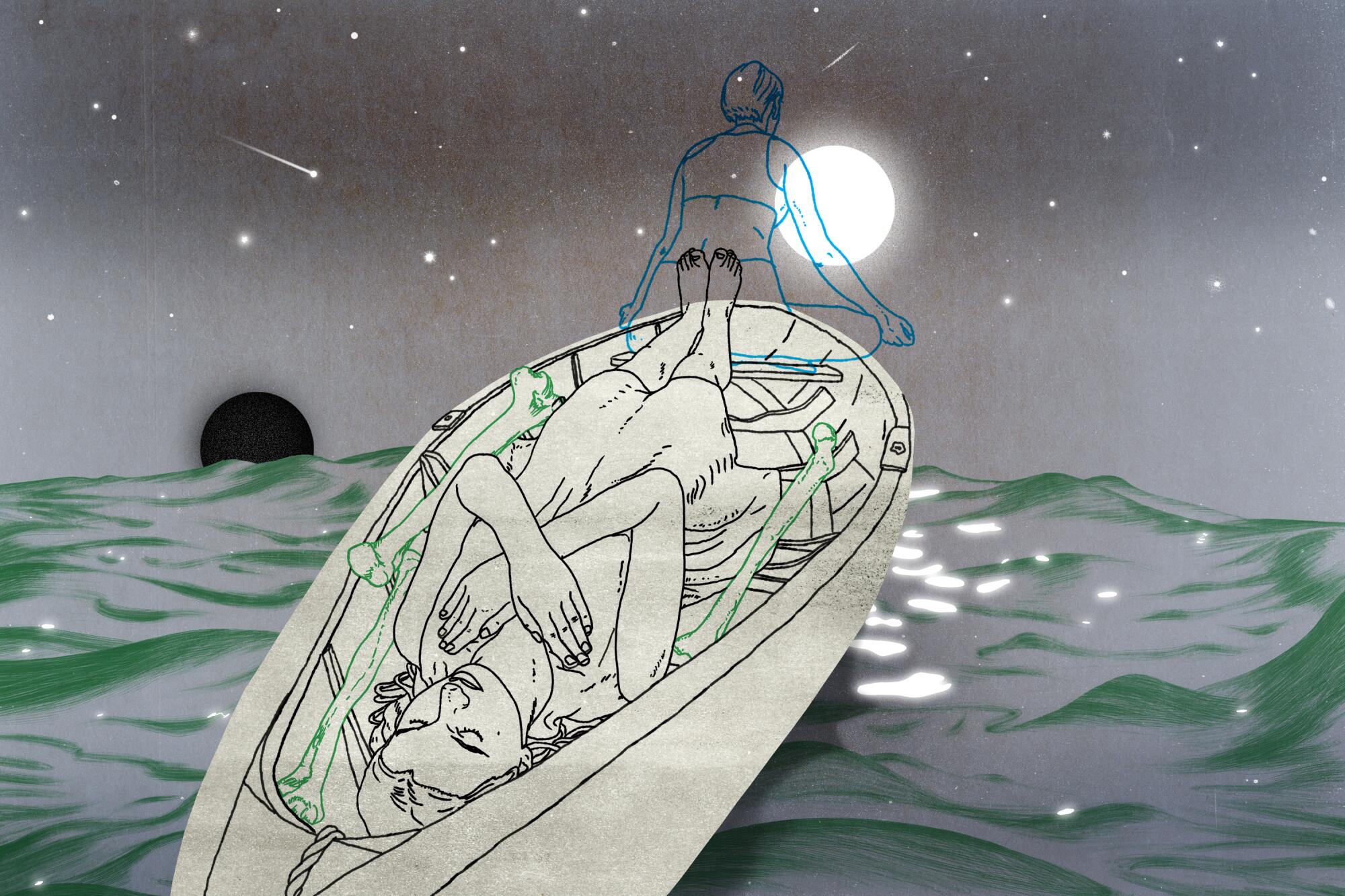The image is a stylized, graphic design drawing depicting a serene yet eerie night-time sea scene. The black night sky at the top transitions into a grayer hue toward the horizon, dotted with small white stars. In the center-right of the sky, there is a large, bright white circle representing the moon, while on the bottom left of the skyline, a prominent black circle, resembling a dark moon, appears to be setting into the ocean. The ocean itself, stretching from the horizon to the bottom of the image, is a greenish color with visible wave strokes.

Dominating the central portion of the composition is the outline of a boat, facing the viewer with its prow slightly tilted upward toward the moon. Inside the boat lies a woman with shoulder-length hair, dressed in a long gown. Her head rests near the bottom of the image, feet pointing upward, and her arms are crossed over her chest in a seemingly peaceful or possibly deceased pose. At the tip of the boat, where it meets the luminous moon, another woman is depicted in a blue outline. She sits cross-legged, facing away from the viewer as if meditating. This woman, dressed in a sports bra and shorts with very short hair, has her arms resting on her knees, complementing the tranquil yet mysterious atmosphere of the scene.